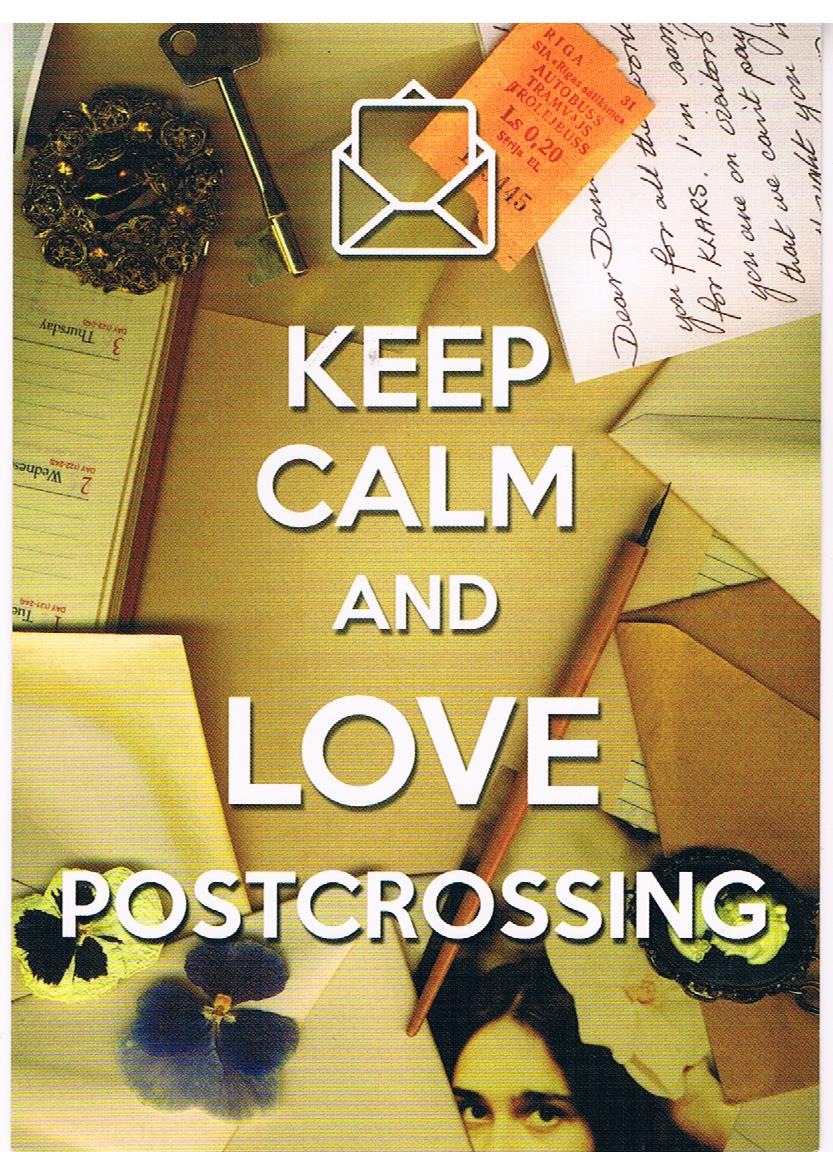The image is a vibrant, full-color postcard with a lot of intricate details. At the very top, there is a logo of an envelope with a document emerging from it, which has a modern, techno feel despite its deliberately yellowed look. Below this, bold white text reads, "Keep Calm and Love Post-crossing," with "Love" and "Calm" being the largest words. On the right side, there is an orange envelope that resembles a seed packet. Next, there's an old-fashioned letter written in right-handed script.

Below the main text, partially obscured, is the face of a young white woman with dark hair, upon which rests an antique ink pen. To the left of her head sits another envelope adorned with a couple of flowers, which appear to be heliotropes, adding a touch of delicacy. On the upper left, there's a vintage book calendar, while the top right features an orange ticket along with a white card bearing black handwriting, starting with "Dear." Scattered around are small objects such as a day planner and possibly a decorative paperweight, contributing to the overall vintage and eclectic desk aesthetic.